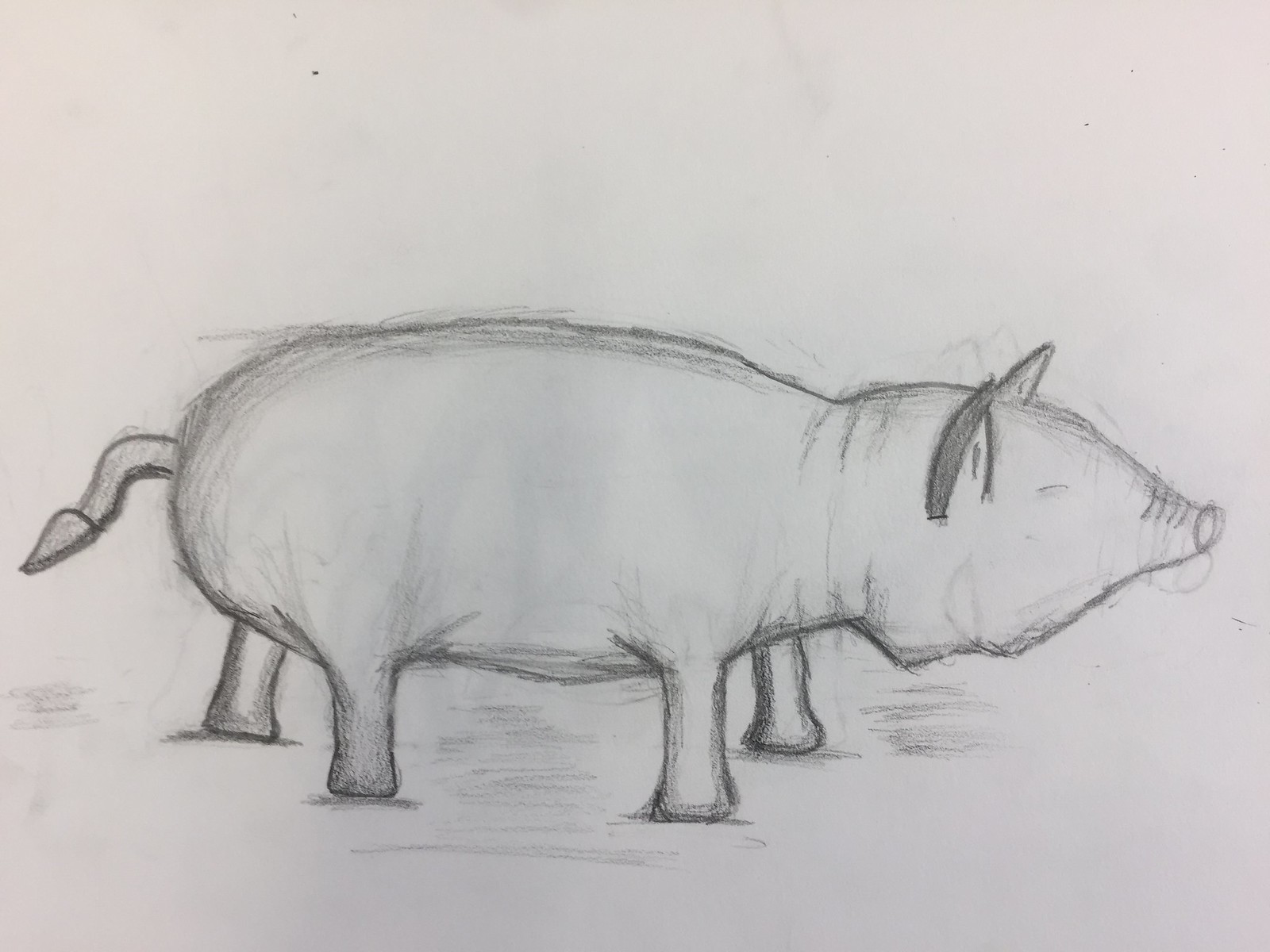This is a monochromatic, pencil-drawn image of a pig depicted in profile, facing to the left. The drawing is on a white piece of paper, and while it isn't highly detailed, it captures the essential features of the animal. The pig's four legs are drawn tapering to stumps rather than detailed hooves. On the left side, the pig's small, curved tail is visible, pointing downward at the tip. On the right, one can see the pig's ears poking up, and a simplistic slit represents the eye, giving the appearance of being closed. Below the pig, the artist sketched some light lines to suggest the ground, adding context to the image. The pig itself is not shaded in but is outlined with pencil to provide some depth, leaving the body largely uncolored.